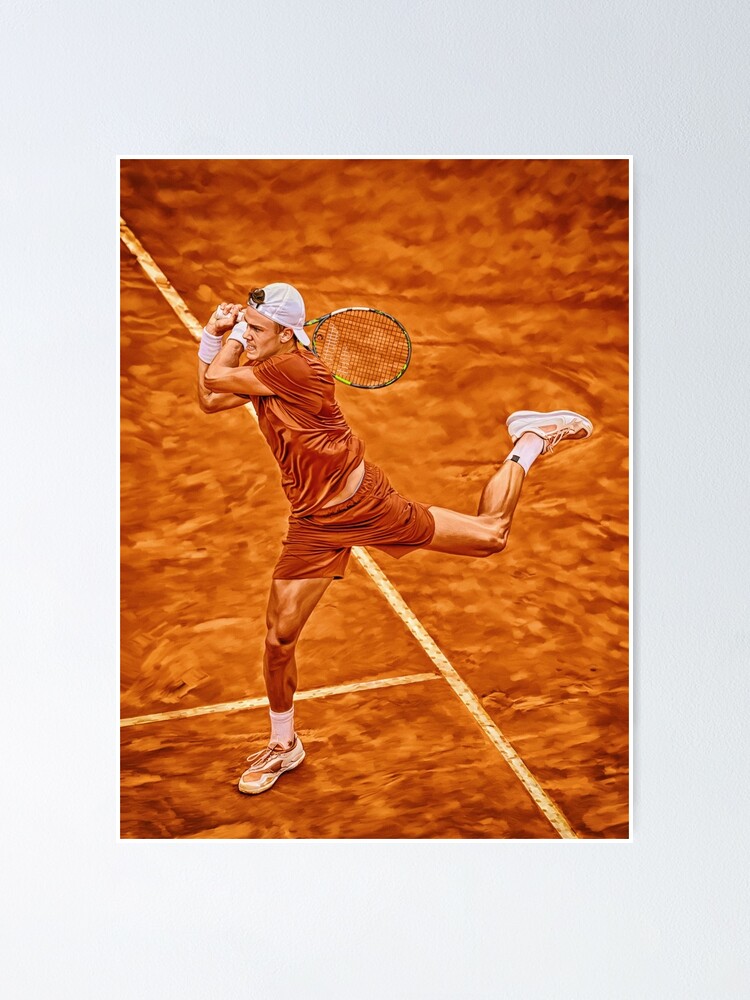A muscular tennis player, deeply focused and exuding seriousness, is captured mid-action on the court. He's clad in a vibrant, orange-colored athletic outfit that accentuates his strong physique. With one leg kicked upward, he appears to be either in the midst of a powerful serve or a dynamic return. The setting contributes to the intensity of the scene, as he plays in a challenging and daring environment that evokes both health and fitness. The court beneath him displays an extensive, marbled pattern, adding an artistic touch to the competitive atmosphere.